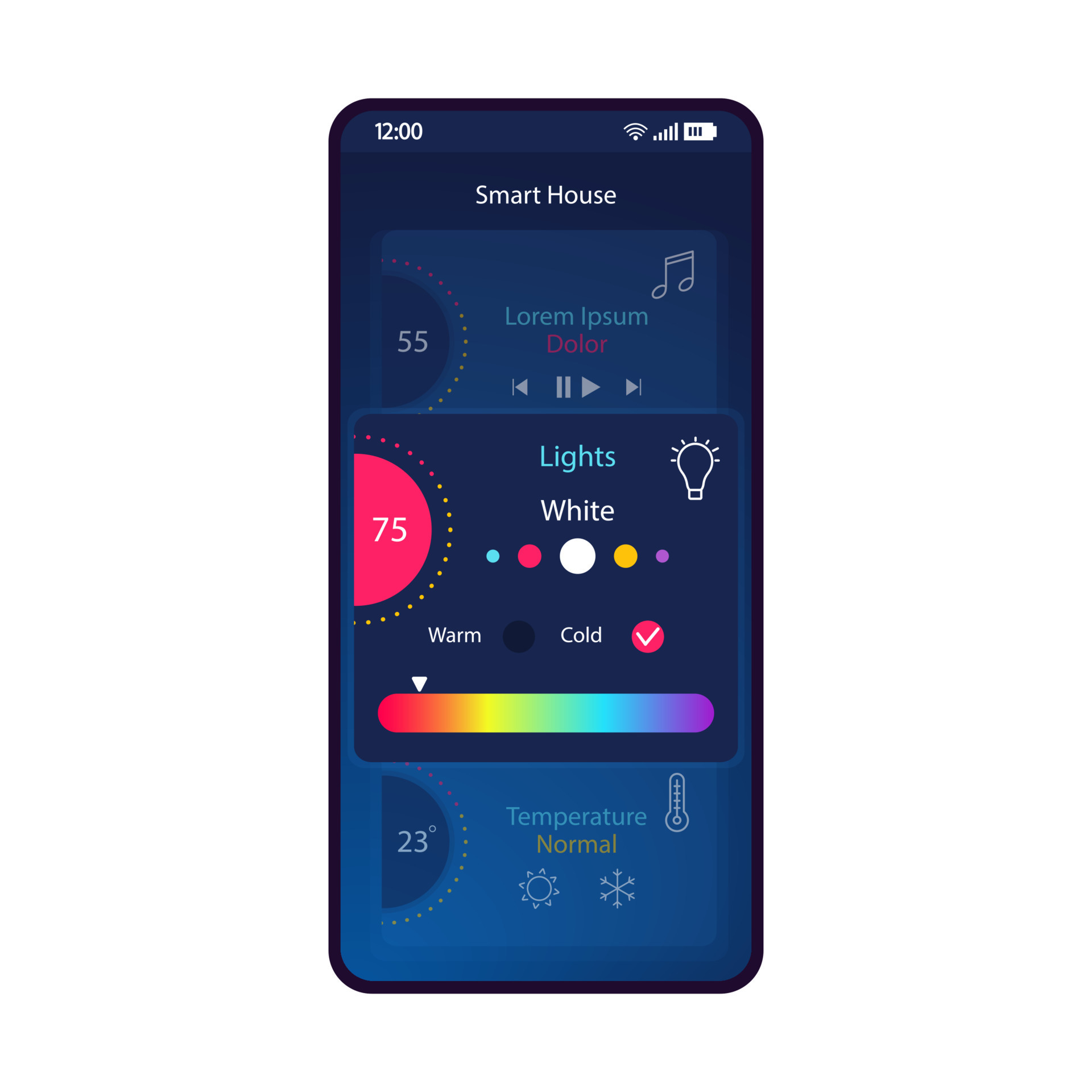The image shows a smartphone screen featuring the home interface of a "Smart House" app, likely used to manage various smart devices within a home. Dominated by a blue background, the screen is divided into three main sections. At the top, there is a music control panel displaying a song titled "Doehler" by the artist "Lorem Ipsum," featuring play, pause, forward, and back buttons for music navigation. The middle section manages smart lighting, currently set to a warm white at 75% brightness. A rainbow-colored hue graph allows users to choose different light tones. On the left side, numerical adjustments are visible, likely representing brightness and perhaps other settings. The bottom section displays the home temperature, set at a comfortable 23 degrees Celsius. This detailed snapshot of the app gives a clear, organized view of controlling music, lighting, and temperature all from a single interface.